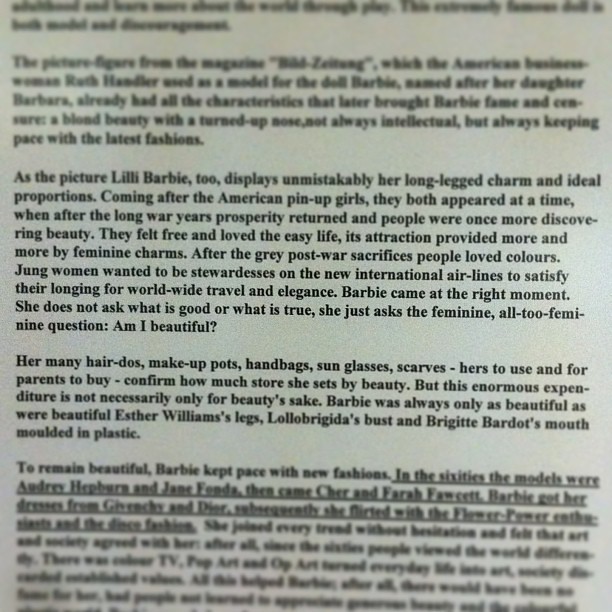This image is a blurry black and white photograph of a page that appears to be cut out from an old, faded newspaper. The page has a grayish background typical of aged newsprint. The layout consists of several paragraphs separated by spaces. Specifically, there are four main paragraphs interspersed with breaks: an initial incomplete paragraph at the top, followed by a legible paragraph mentioning Lily Barbie's long-legged charm, another space, and then a paragraph discussing Barbie's beauty attributes in comparison to famous figures such as Esther Williams, Lola Bridget, and Bridget Bardot. The lower end of the page features another incomplete, blurred paragraph. Despite the overall poor legibility and the dirty, deteriorated condition of the print, it's evident that the article is about Barbie and her iconic beauty as represented in popular culture.